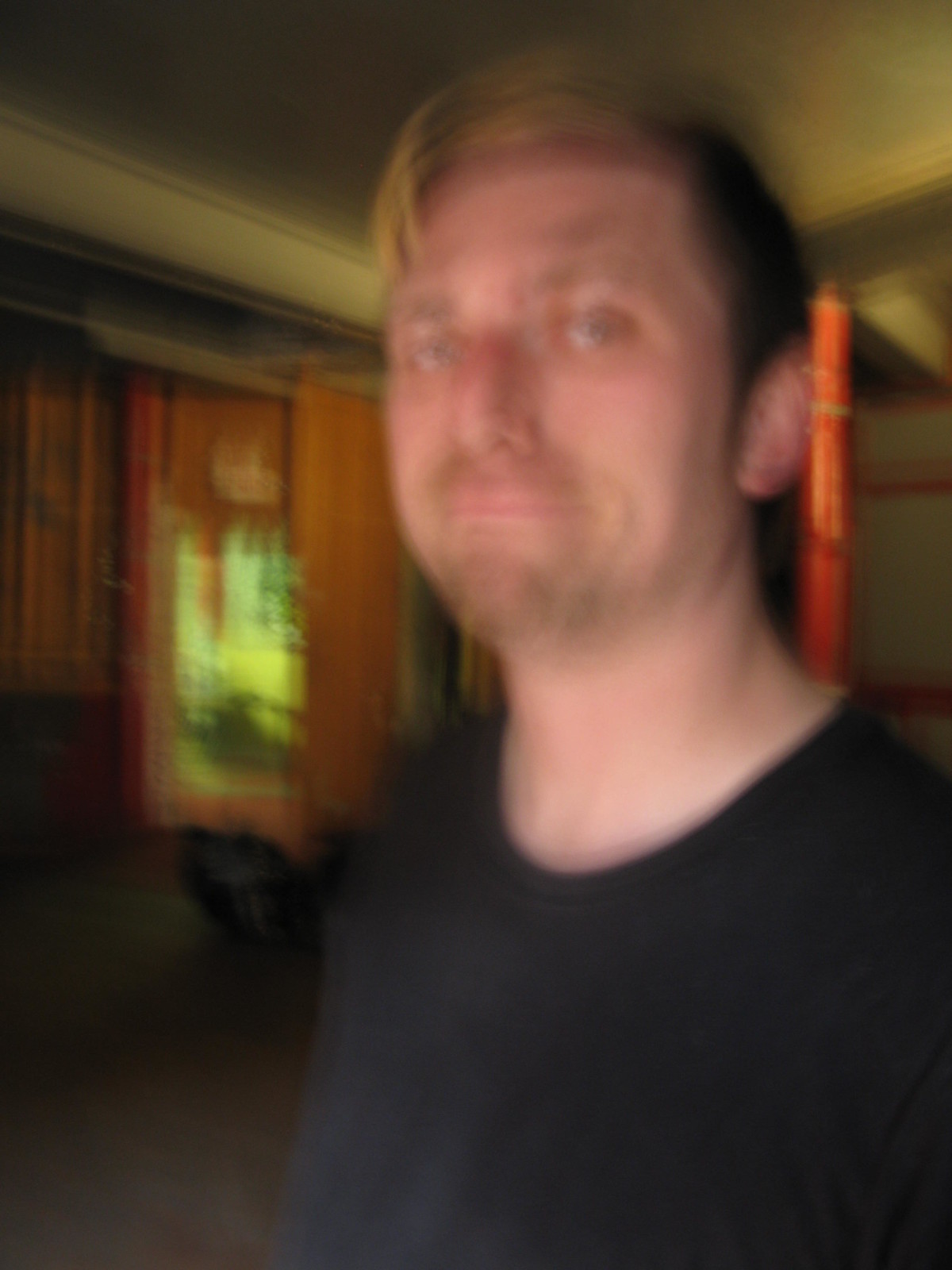A somewhat indistinct image captures a man standing inside a house. Though blurry, the man is discernible, appearing slightly clearer than the background. He is dressed in a black shirt and is positioned with his body angled toward the lower left, while his face is turned toward the camera. The man's facial features include a goatee-like beard, blonde hair, and what seem to be blue eyes. The background is even more blurred, but it reveals a wooden wall and a window partially covered by red curtains. The overall quality of the image is low.